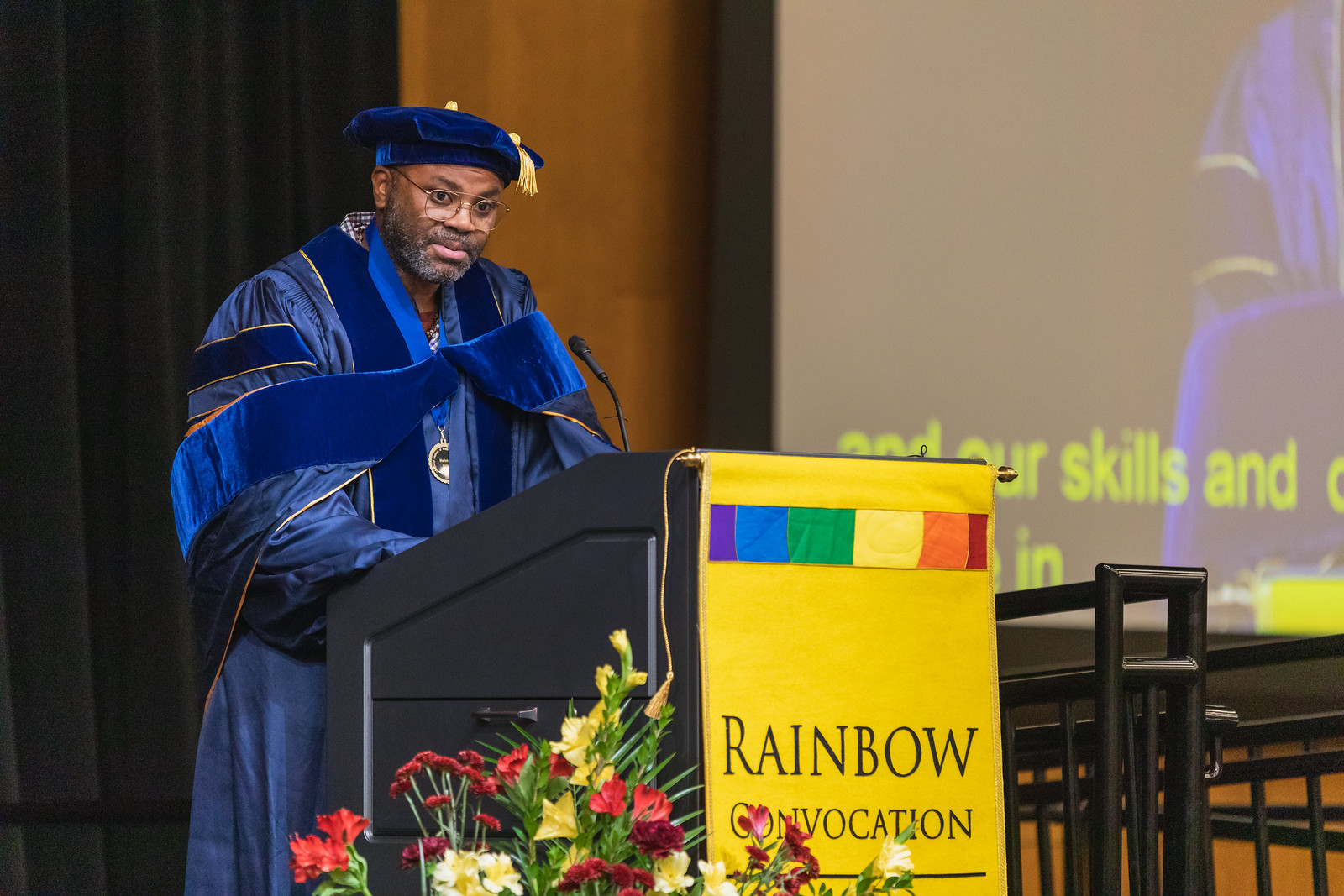The image captures a distinguished African-American man at a podium during a graduation ceremony, likely a college convocation. He is dressed in an ornate blue Ph.D. cap and gown with blue velvet details and a gold tassel, giving him an air of academic distinction. The podium, which is black, is adorned with a yellow banner that reads "Rainbow Convocation" in black letters, topped by a small rainbow illustration. At the base of the podium, red and yellow flowers add a touch of color to the scene. In the background, a large projection screen displays a live feed of the speaker, with yellow closed captions transcribing his speech. His salt-and-pepper beard, mustache, and glasses contribute to his scholarly appearance as he addresses the audience, facing diagonally to the right.